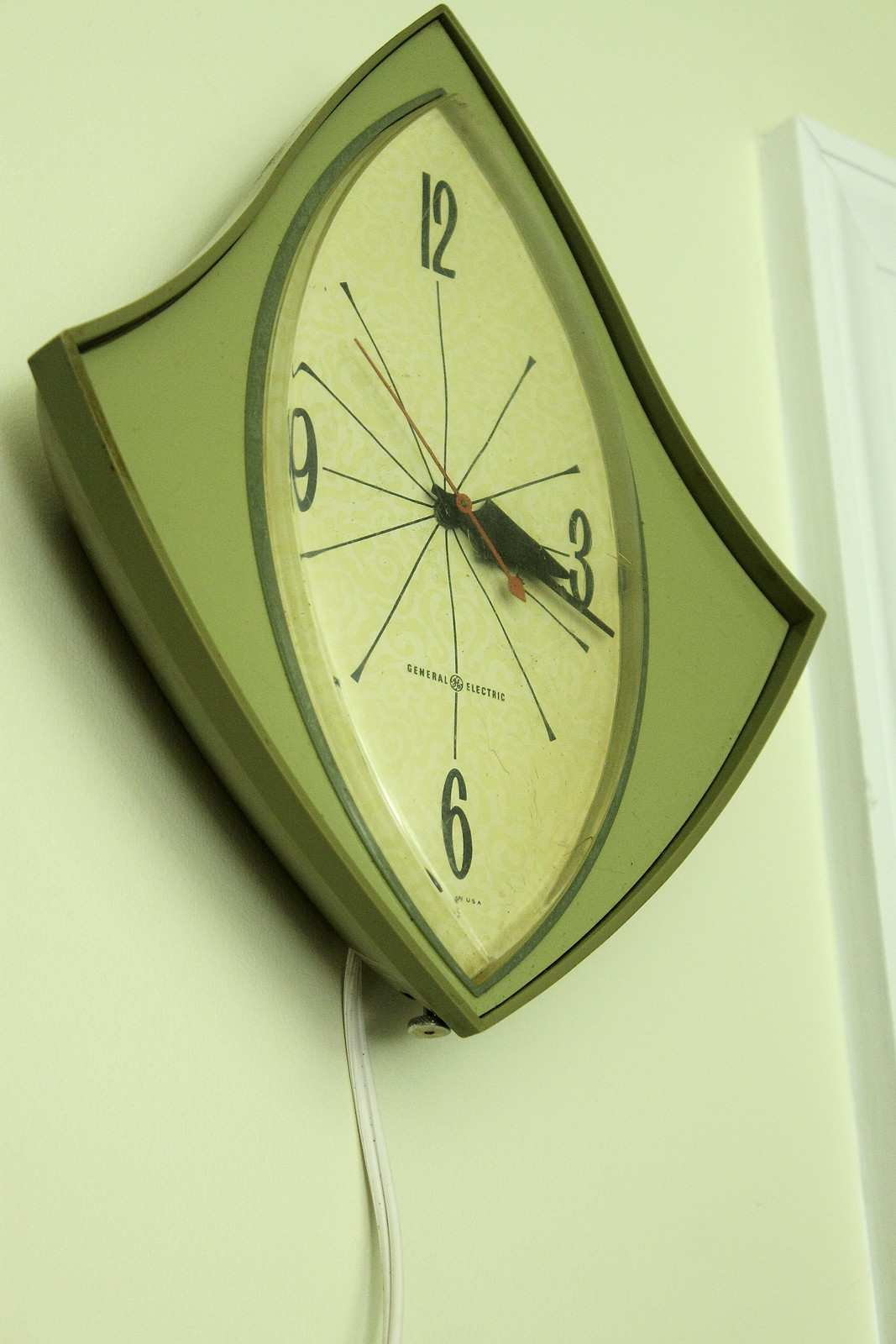This photo features a uniquely shaped wall clock that bears a resemblance to a stingray or an oblong diamond with pointed ends. The clock, predominantly a sage or olive green, has a darker green rim around the face, creating a layered effect with the lighter hue inside. The clock face prominently displays the numbers 12, 3, 6, and 9 at the cardinal points, with two tick marks between each pair of numbers, deviating from the design of a standard clock. The clock hands are distinct, with the hour hand being thicker, the minute hand thinner, and a red second hand adding a vibrant contrast. Below the clock, a white power cord hangs down and continues off the edge of the frame. The clock is mounted on a very light green wall that complements its color scheme. On the right-hand side of the image, a white door frame is partially visible, further framing the clock as the focal point of this scene. The brand "General Electric" can be read on the clock's face, adding to its character.